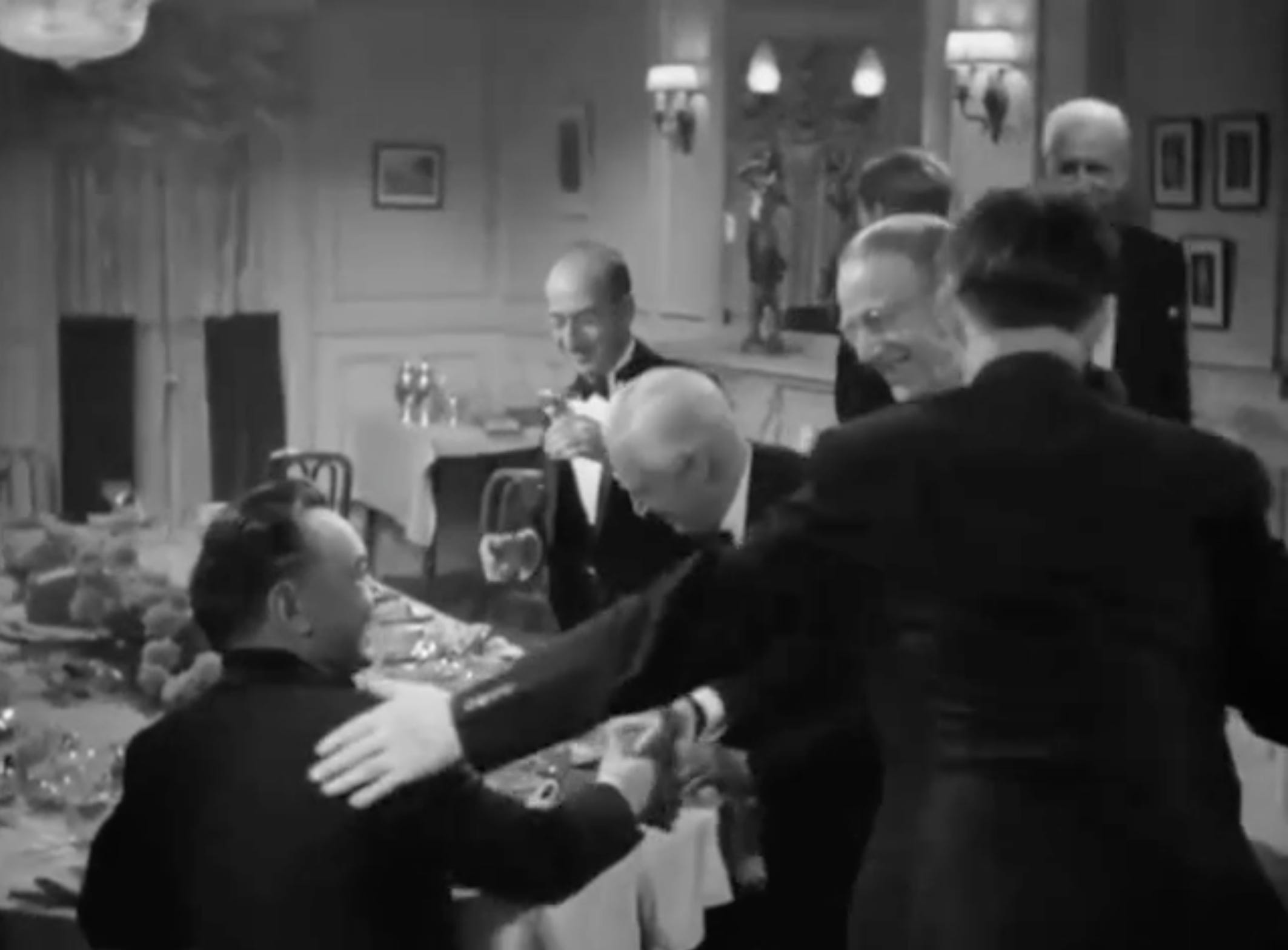This black-and-white photograph, likely taken in the 1930s or 1940s, captures a lively dining room scene featuring seven formally dressed men in black suits or tuxedos, several of whom have short or slicked-back hair. At the head of a dinner table set with cutlery, dishes, plates, and glasses—possibly filled with champagne—sits an older gentleman, the focal point of the gathering. He is seated in the foreground, with another man to his right, affectionately placing a hand on his shoulder, while another bends over, perhaps to shake his hand, and other men stand around laughing and holding glasses. The backdrop includes richly detailed wooden walls adorned with paintings, framed pictures, and elegant light fixtures. Curtains suggest a door to the side, and on the back wall, additional glasses are visible on a table, underscoring the convivial atmosphere of the scene.